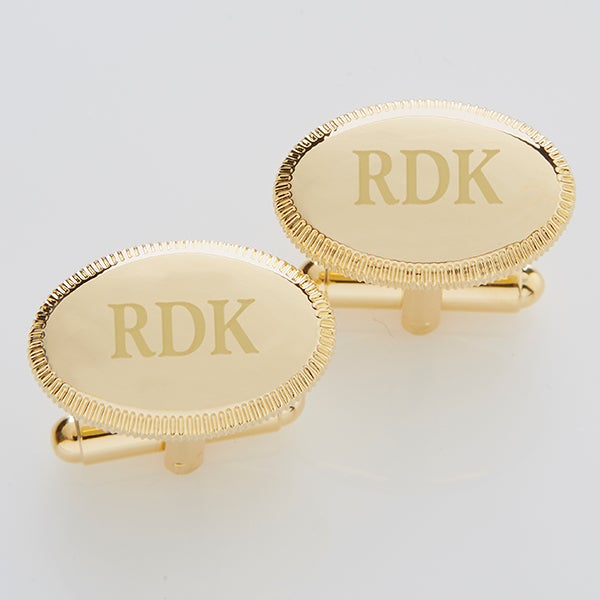This close-up image shows a pristine pair of oval gold cufflinks against a bright white background. The cufflinks prominently feature the monogram "RDK" etched into the center of each piece. They have a polished appearance with light reflecting off their surface, highlighting the lustrous golden hue. Surrounding the monogram, each cufflink displays a serrated perimeter, giving it a distinguished and detailed border design reminiscent of outward-facing 'U' shapes akin to paper clips. The cufflinks appear to be brand new and are placed in such a way that one is positioned slightly above and to the right of the other. The setting is minimalistic, with no additional elements in the background, accentuating the elegant and vivid display of these sophisticated accessories.